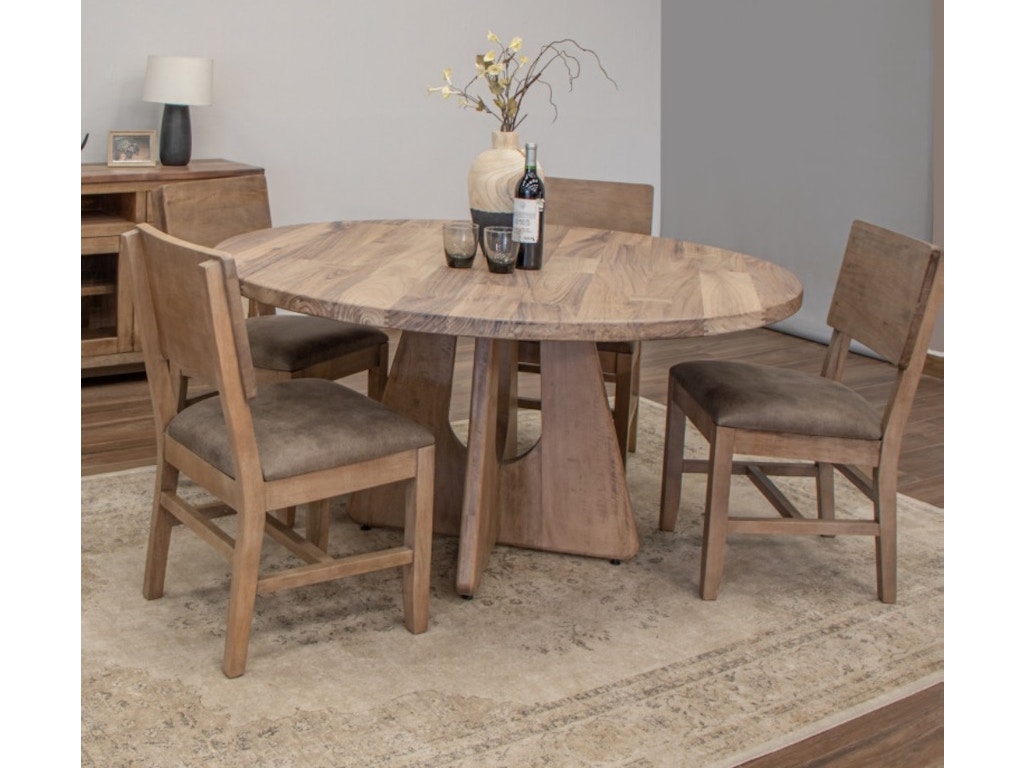This photograph captures a cozy dining or kitchen room setting centered around a round, light wooden table with a distinctive intersecting triangular base. Surrounding the table are four matching wooden chairs, each adorned with brown cushions. The table is set on a beige, printed rug that lies on medium brown hardwood flooring. Central to the scene, the table holds a bottle of wine and two short glasses, along with a wooden jug-style vase filled with twigs and yellow flowers.

In the background, against the light gray wall to the left, stands a wooden cabinet that doubles as a bookshelf or counter, featuring a lamp, a framed picture, and two windows on its lower portion. The walls in the room are painted in shades of gray, contributing to the serene and inviting ambiance of the space. Overall, the image evokes a sense of warmth and hominess, blending simple, rustic furniture with subtle decorative touches.